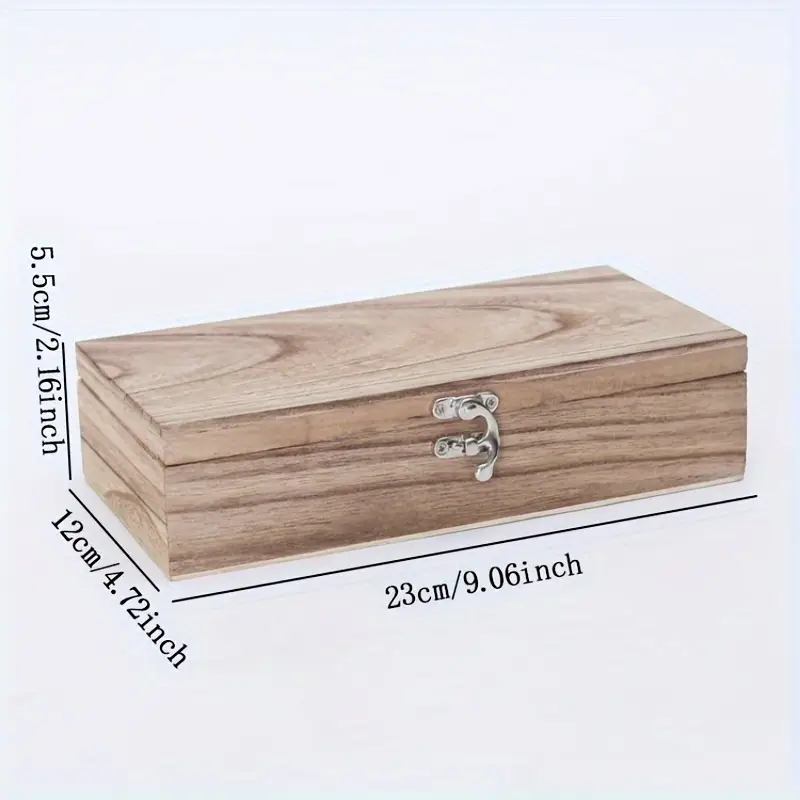The photograph features a natural light wood grain rectangular box with no stain or finish, set against an off-white background. The box, resembling the style of a jewelry box, prominently displays its dimensions with black measurement lines: 23 centimeters (9.06 inches) in length, 12 centimeters (4.72 inches) in width, and 5.5 centimeters (2.16 inches) in height. Attention is drawn to the silver latch on the front, which has a functional two-piece mechanism involving a lever that slides to the right and spins upward to release from a loophole, securely closing the lid. The latch is detailed with two screws on both the upper and lower parts, contributing to its secure closure. The image is devoid of any other elements, highlighting the intricate texture and grain of the wood, suggesting an advertisement focus for the box.